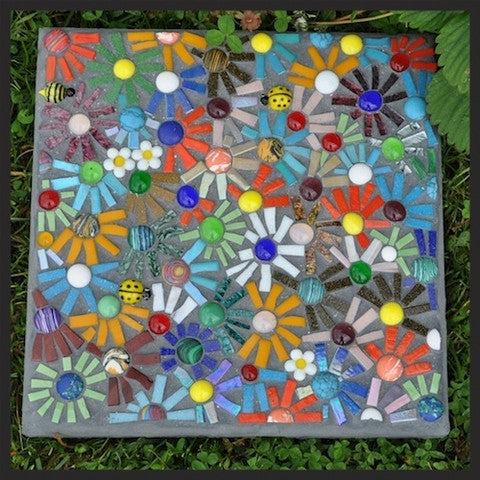The image captures a piece of vibrant and intricate artwork resting on a gray square paver stone, likely made of concrete or a similar material, situated on a bed of green grass and surrounded by lush, green leaves and clovers. The artwork itself is composed of multicolored, ceramic-like pieces arranged in various shapes and patterns. Prominent among these are several depictions of the sun, with colorful rays radiating outwards from central circles, painted in hues of green, yellow, turquoise, blue, and red. One notably detailed part of the artwork features a yellow and black striped bumblebee in the upper left corner and, somewhat incongruously, a ladybug. Surrounding these central images are additional circular and rectangular shapes in various colors such as white, purple, orange, and dark blue, mimicking the look of flowers and adding to the mosaic-like aesthetic of the piece. The array of colored tiles and painted elements give the artwork a rich, decorative quality that stands out against the natural background.